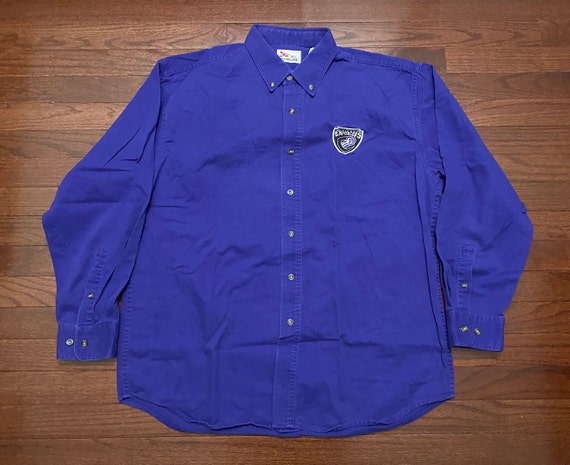This image showcases a men's royal blue, long-sleeve, button-down shirt with a button-down collar, meticulously laid out on a wooden floor, which has some marbleization patterns. The shirt features silver buttons down the middle, including buttoned cuffs on the sleeves, which are neatly folded in the same manner. The shirt appears to have creases and wrinkles, suggesting it needs ironing. On the left chest area, there's a small shield-shaped patch that is black with some white writing and an emblem, indicating it might be a company shirt. The shirt's label is visible beneath the collar but illegible. The overall impression is of a well-kept, slightly worn shirt, potentially being resold, with the details presented clearly against the wooden floor background.